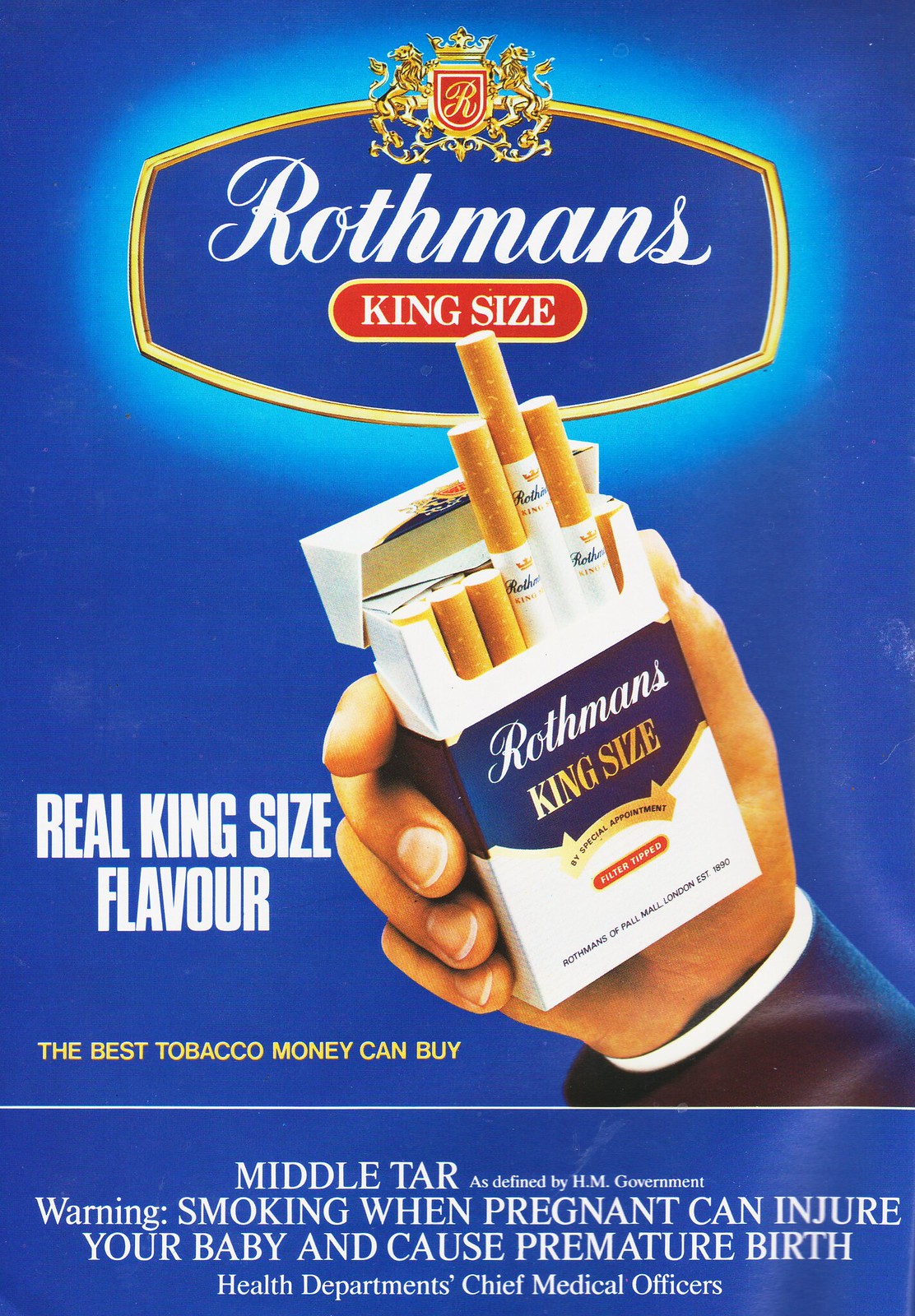The image is a computer-generated advertisement poster with a blue rectangular background, longer in length than width. The focal point of the image features a man's hand holding a white cigarette pack with a dark brown middle section prominently displaying the text "RUVEMENTS KINGSIZE." Above the pack, a logo is situated at the top of the image, consisting of two parallel lines with a red seal in the middle, containing the letter "R." Below the logo, the brand name "RUVEMENTS" is written, followed by "KINGSIZE." To the right of the cigarette pack, the text reads "REAL KINGSIZE FAVOR." Additionally, towards the bottom, more text appears, including a health warning that states: "Medaltar as defined by HM Government: Warning, smoking when pregnant can injure your baby and cause premature birth. Health Department's Chief Medical Officers." This detailed composition and specific branding elements make the advertisement visually compelling and informative.